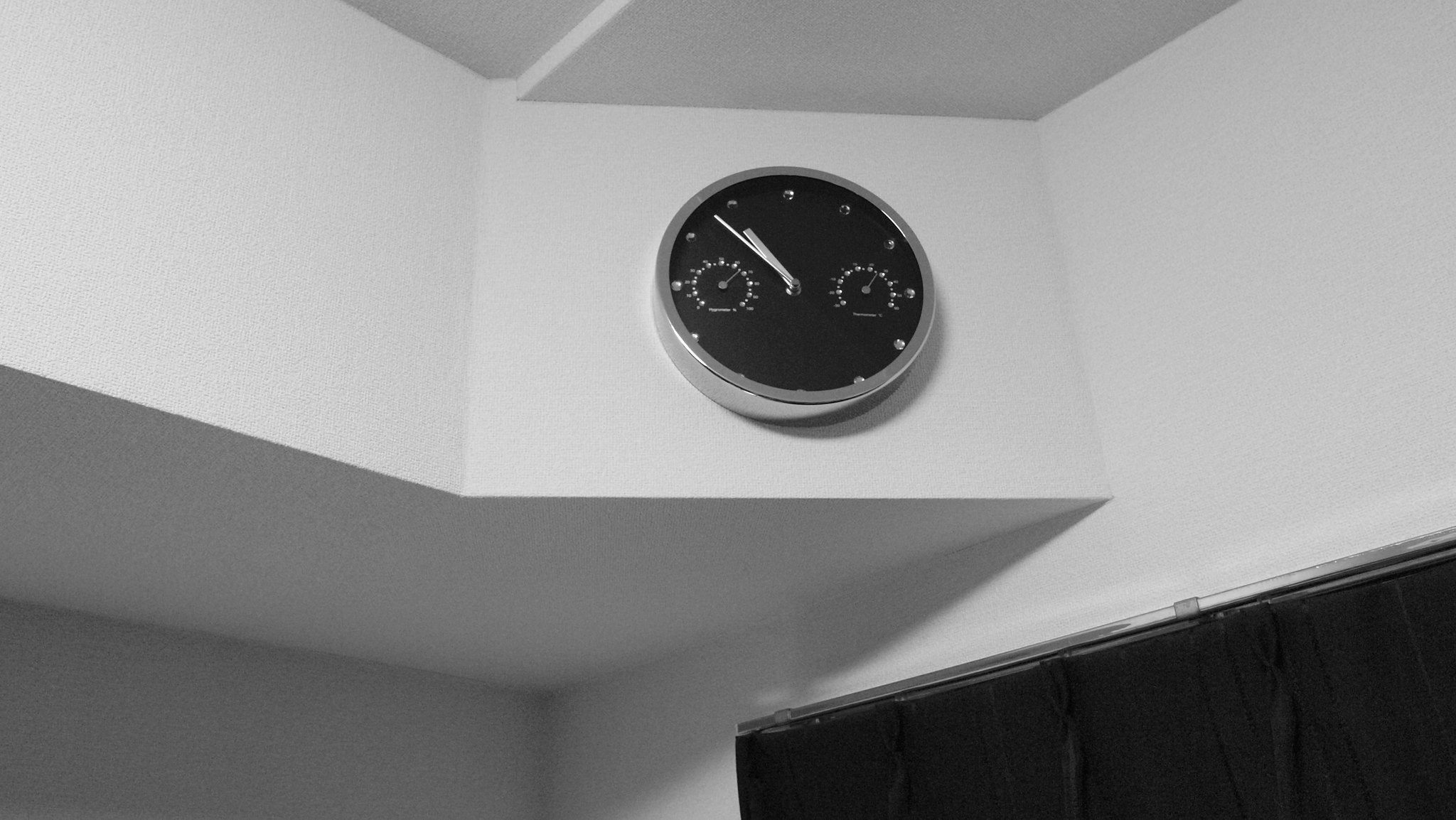This photograph captures the interior of a modern building, showcasing a sophisticated room designed in a monochromatic palette of black, white, and shades of gray. The walls are painted in a light gray or white, contributing to the sleek ambiance of the space. 

The focal point of the image is an elegant clock mounted on a jutting structure resembling an awning. The clock itself is black with a striking silver outline. It features a pair of silver hands and is adorned with either dots or jewels in place of traditional numbers. This design adds an element of luxury and uniqueness to the timepiece.

Flanking the main clock are two smaller clock faces, likely designated for seconds or other specific measurements of time. Adding to the room's modern aesthetic, a large black curtain is partially visible, hanging on the right side below the central clock. The combination of these elements creates a refined and contemporary atmosphere within the building.